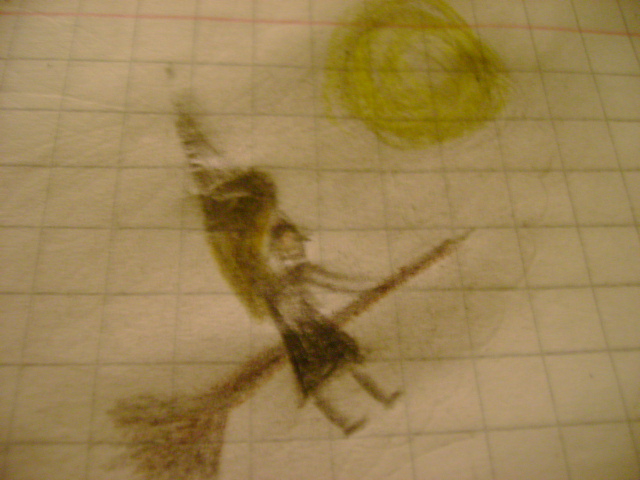This image appears to be a child's crayon drawing on white graph paper, characterized by a single horizontal red line at the top. The central focus of the artwork is a witch, depicted with long black hair, a black pointy hat, and a black dress. The witch is sitting on a diagonally-oriented brown broomstick, suggesting she is flying. A prominent yellow circle, likely representing the moon, is located near the top right of the image. The graph paper's light gray grid is evident throughout. Overall, the drawing is simple and whimsical, embodying the playful, imaginative style typical of children's art.